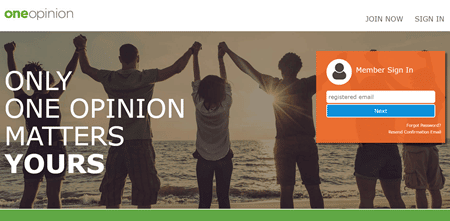Screenshot of One Opinion website: The website features a sepia-toned background photograph of children standing on the shore of a lake or ocean, bathed in the soft light of a setting sun. The children, dressed in casual attire, are holding hands and raising them high in united exuberance, facing towards the west. Prominently displayed in the center of the page, the main headline boldly declares, "Only One Opinion Matters. Yours." To the right of this headline, a pop-up box prompts users to either join now or sign in by entering their registered email, effectively guiding them to the next step. Grounding the entire page, a very thin green bar lines the bottom, echoing the same hue used in the 'One' of the One Opinion logo, adding a touch of cohesiveness to the page's design.